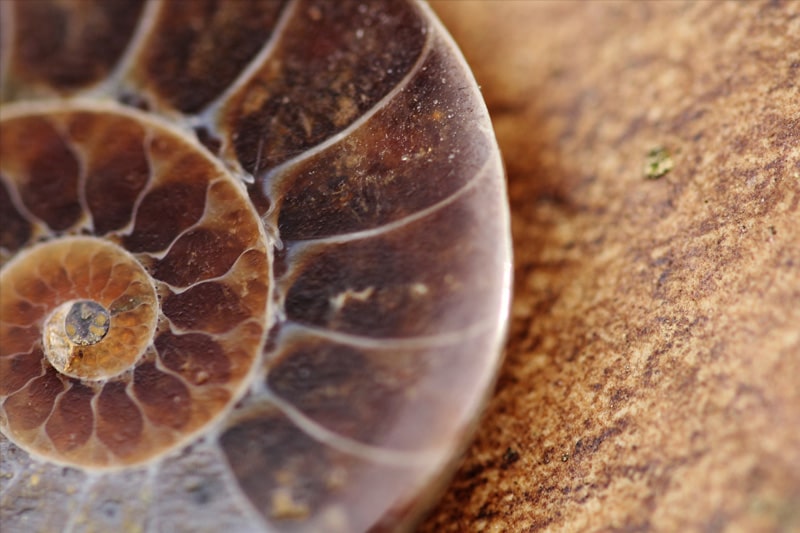This close-up underwater photograph features a brown spiral shell, likely of a mollusk or snail, situated on the left side of the image. The shell exhibits a curling, cinnamon roll shape, with its various chambers segmented by white lines. The predominantly brown shell is lighter on the right side, possibly due to sunlight, and also shows white flakes and scratches, indicative of either natural markings or minor damage. The image reveals a portion of the inner chamber where the exterior appears to have broken off, exposing white areas beneath. The shell's intricate details blur towards the edges, particularly along the left. The right side of the photograph captures a sandy surface with visible individual grains, interspersed with black and green flecks. A shadow cast by the shell darkens part of this sandy expanse, highlighting the shell's presence in the otherwise muted underwater landscape.